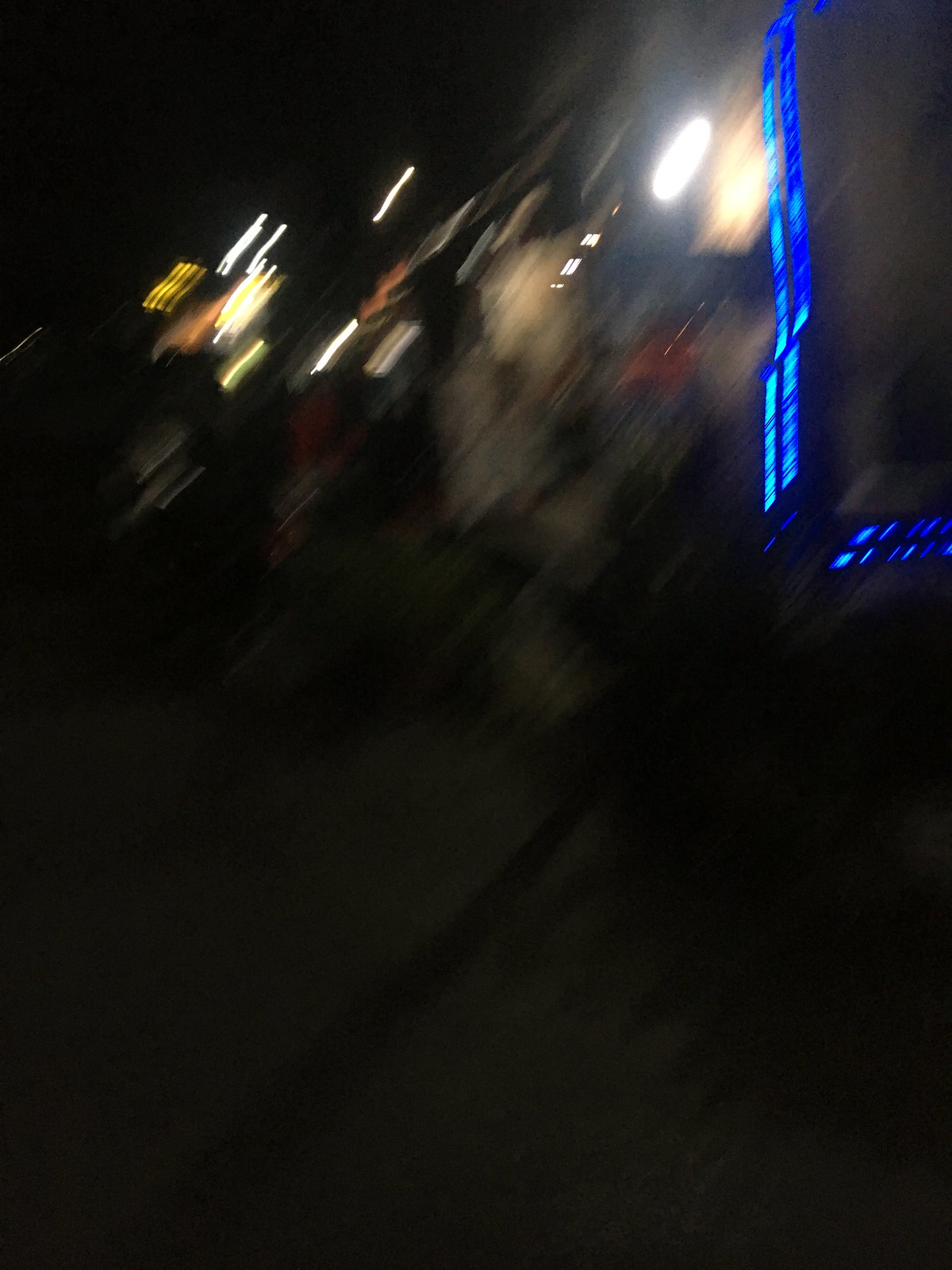This is an extremely out-of-focus and blurry vertical rectangular photograph taken at night. The upper left-hand corner is completely black, gradually shifting to a slight grayish hue with some green and red discoloration. The right side of the top edge features a prominent, double blue vertical light resembling a neon strip, extending down to about the halfway mark. In the upper right-hand portion, a streak or slashes of blue light can be observed next to some oval-shaped white lights. Scattered throughout the image are worm-like streaks of various colors, including yellow, white, blue, and orange, creating a smoky effect where the colors bleed into each other. In the center, slightly higher than the middle, there is a noticeable blur, accentuated by a big circle of light causing glare, making it difficult to discern any recognizable objects. The bottom of the image remains dark, with faint shadows visible.